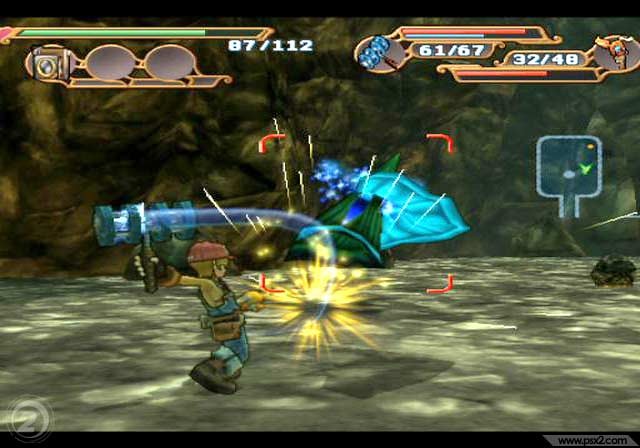This is a vibrant screen capture from a computer game or console, featuring a dynamic scene with a vivid green and yellow smudge-like background. In the foreground, a blend of light green and yellowish-white smudges create a luminous surface. Positioned to the left, a character is depicted in a dramatic pose, leaning backward with one arm extended behind him, grasping a hammer-like tool raised above his head. His left foot, bent at the knee, juts out to the side, adding to the sense of action. 

The character is dressed in a yellow shirt paired with blue jean overalls and sports a red cap atop his head. His light hair and fair skin complement the ensemble, which is completed with a tool belt slung around his waist. From the hammer-like tool, he is emitting a radiant beam of light, and a shower of yellow sparks cascades in a circular pattern onto the ground ahead of him, emphasizing the intensity of the scene.